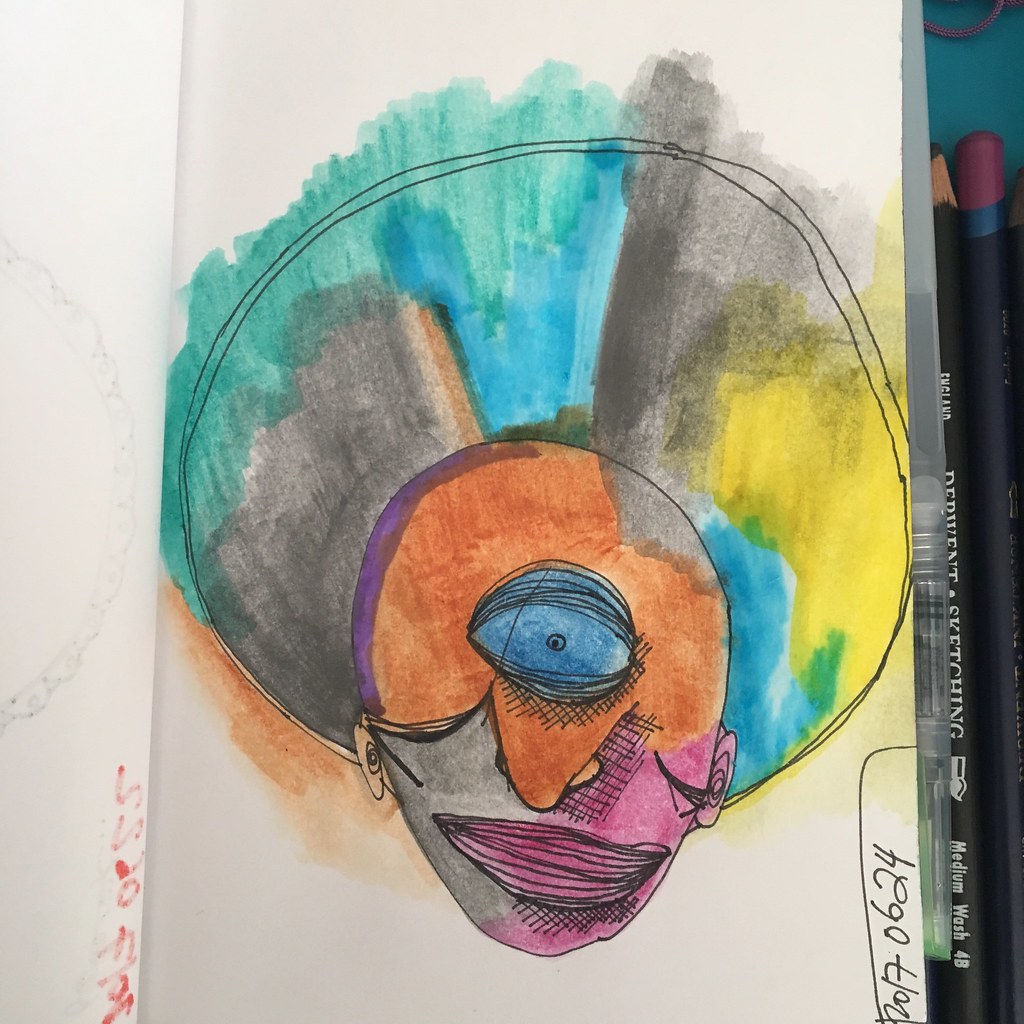The photograph showcases a captivating watercolor painting on white paper. The left edge of the painting is unmarked, while the right edge features a black pole capped with maroon and a hint of blue beneath it. Central to the painting is a stylized head, vividly outlined in black with a rounded top tapering into a narrow chin. Dominating the center of the face is a striking blue oval eye, characterized by a black iris with a pinpoint black pupil and accentuated by sleek, curved lines that form a lid. 

The upper portion of the head is painted in a bold orange, contrasted by a delicate purple outline on the left side and a small gray square in the upper right corner. The orange hue continues beneath the eye, extending into a pronounced V shape. The lower left portion of the face transitions into gray, while the lower right area is painted in a soft pink. A prominent, thick pink mouth sits widely on the face, adding to the expressive nature of the painting.

Each side of the head features ears positioned naturally, from which circular shapes emerge and ascend. These circles are filled with a vibrant mix of colors: the right circle blends yellow, blue, and gray, while the left circle transitions from orange at the bottom to gray and then blue as it ascends. This detailed and dynamic composition highlights the artist's innovative use of color and form, making the watercolor a striking and thought-provoking piece.